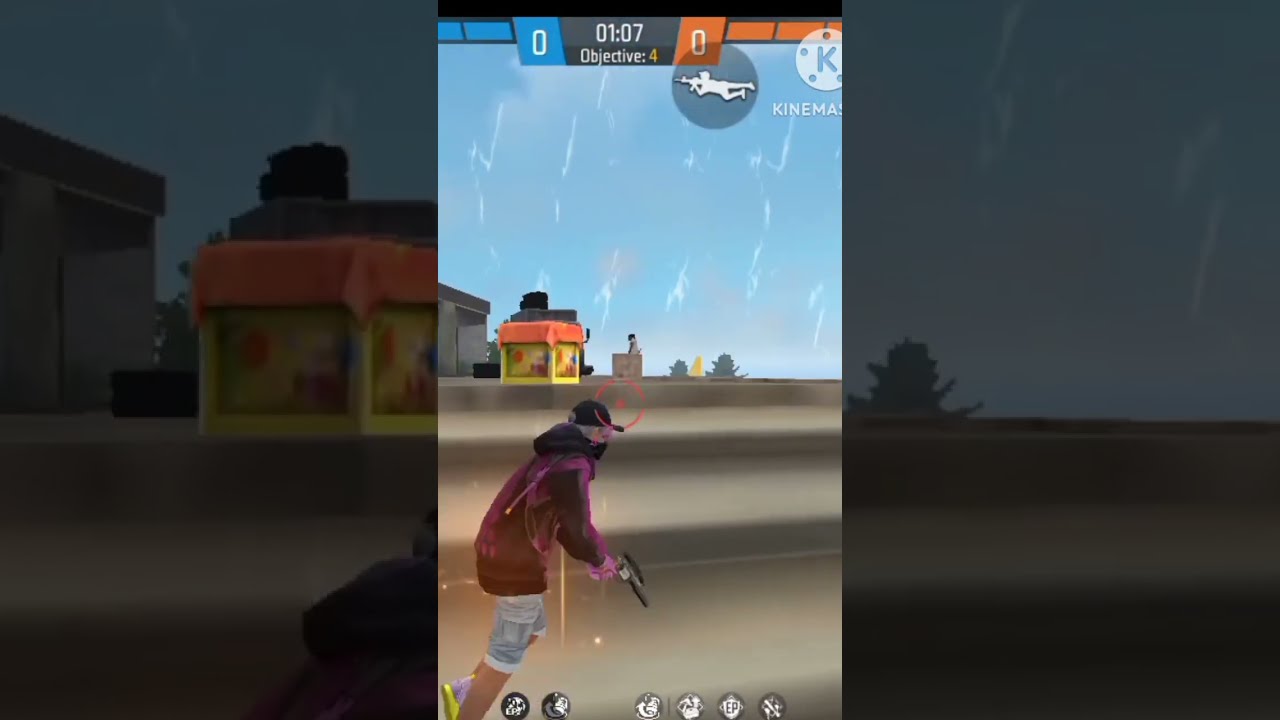The image is a rectangular, horizontal screenshot from a third-person video game divided into three panels. The left panel is darkened, showing a nighttime scene with a fragment of the sky at the top, a building with a pink awning beneath it, a pile of tires, and another building with a chimney. A street runs along the bottom, partially visible. The middle panel is clearer and brighter, predominantly featuring the game's graphical user interface: a top strip displaying a score (0 in blue), a clock reading 0107, the word "Objective" followed by a partially visible "4," and another score (0 in red) with bars. Below this, a circle with an image and a light circle with a K surrounded by dots are shown. This panel also displays a yellow building with a red roof and chimney, part of a gray building to the left, and additional indistinct structures to the right. The scene includes a street and at the bottom, a white male character with a baseball cap, brown jacket, purple splotches, gray shorts, and a gun aimed downward in his right hand. Six circles with icons are displayed along the bottom. The right panel, also darkened, features a sky seemingly in rain and a structure fading into the background. A brown street finishes the lower portion, transitioning from lighter to darker brown. The overall background frames the same city scene, zoomed in and faded out, emphasizing the gold-yellow building with a reddish roof and the expansive sky.